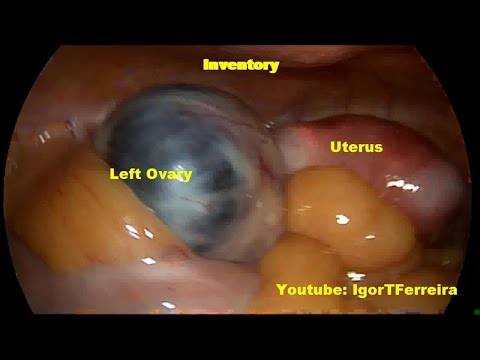This is a detailed, color photograph of the internal female reproductive organs, displayed against a solid black background. The central focus of the image is a mix of vibrant colors showcasing the anatomical structures. At the top, in yellow text, the word "Inventory" is prominently displayed. Below this, the left-hand side features a pink and orange region with a dark, rounded mass identified as the "left ovary" in yellow letters. The center of the image contains a bluish-black, white, and pink spherical object. On the right-hand side, there's a large, shiny, pink-red area labeled as the "uterus" in yellow text. In the lower right-hand corner, the text "YouTube: Igor T. Ferreira" is displayed. The anatomical details appear as if captured through an inserted scope, providing an intimate, close-up view of the female reproductive system.